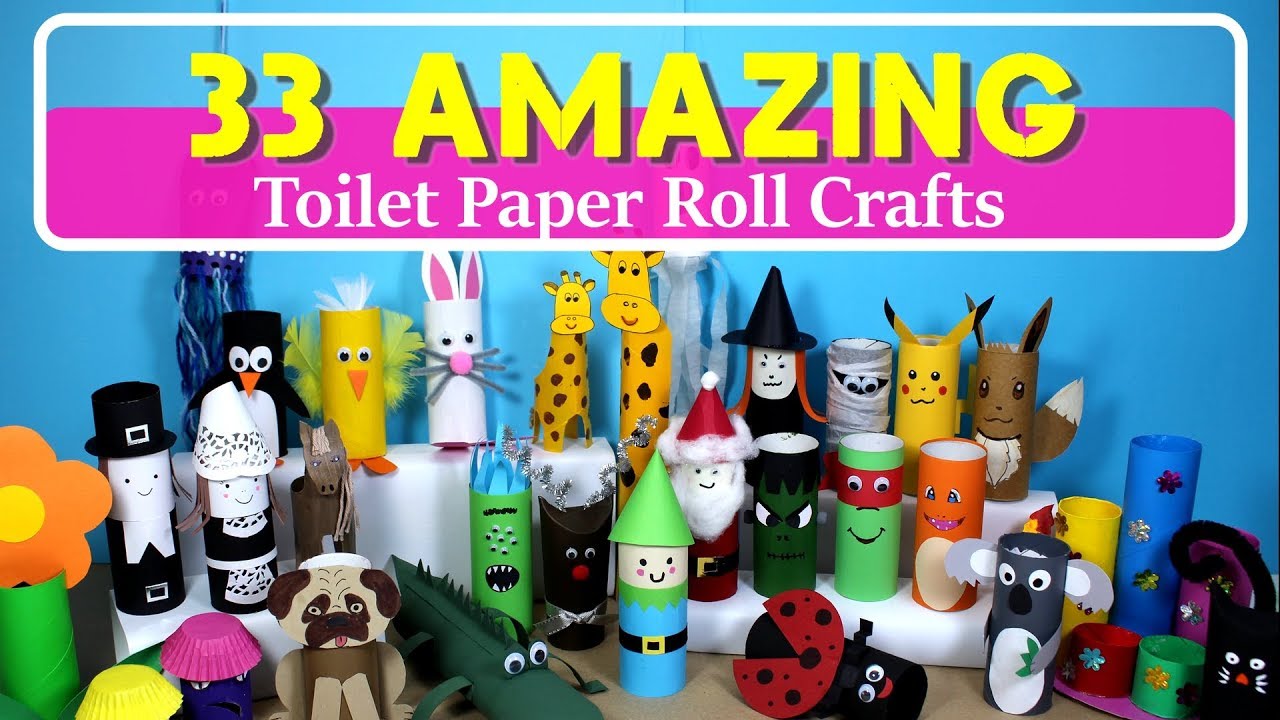The image is a digital photograph of a tan table against a blue wall, showcasing various DIY toilet paper roll crafts. A prominent rounded rectangle with a white border sits at the top, featuring large yellow text with a gray drop shadow that reads "33 Amazing," and smaller white text underneath that says "Toilet Paper Roll Crafts." Below this banner is a magenta color block that extends about two-thirds of the way up. The table is covered with creatively crafted toilet paper rolls transformed into an array of characters and objects, including pilgrims, penguins, birds, a pug, an alligator, Santa, the Incredible Hulk, Raphael from the Teenage Mutant Ninja Turtles, Charizard, a koala, Eevee and Pikachu from Pokemon, a mummy, a witch, two giraffes, a bunny, a ladybug, a cat, flowers, and possibly some jellyfish. The crafts are painted and decorated with a variety of colors, including black, green, gold, red, blue, yellow, purple, pink, and brown, making for a vibrant and imaginative display.